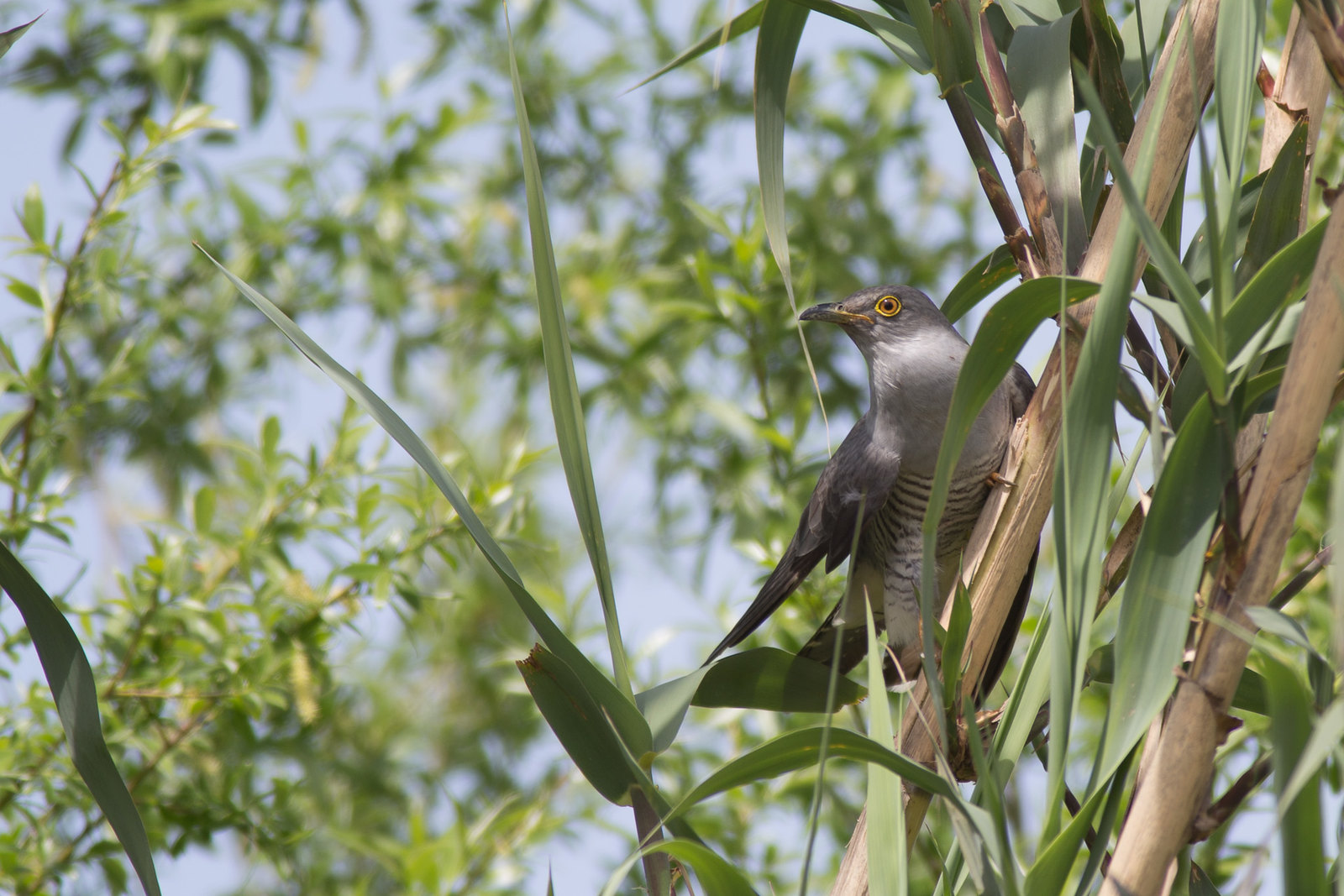The photograph, taken outdoors during the daytime, captures a striking Himalayan cuckoo perched on tan-brown reeds resembling bamboo, amidst lush prairie grasses and foliage. The rectangular image, wider than it is tall, showcases the bird with its head turned left, revealing a distinctive yellow eye with a black center. The bird displays an elegant contrast of darker gray wings against a silver-gray body, adorned with a conspicuous black horizontal stripe on its light gray abdomen, extending to its upper legs. Its wingtips and long tail are outlined with precision, further enhancing its majestic appearance. The cuckoo's black beak, encircled with yellow at the base, and its yellow claws add to its distinctive charm. The background blurs into a serene mix of green leaves and bright blue sky, drawing the viewer’s focus to the bird perched gracefully on the slanted reed, looking vividly alive amidst the soft, blurred foliage.